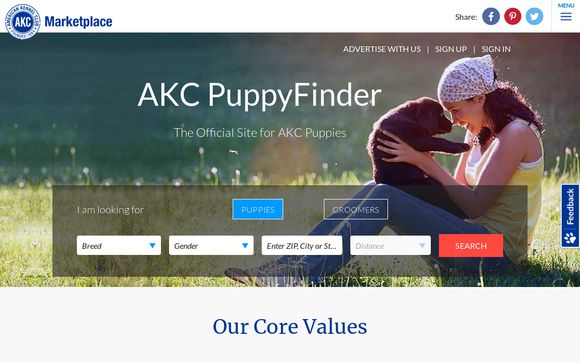This image is a screenshot of a website for a kennel club, specifically the American Kennel Club (AKC) Puppy Finder. Dominating the center of the page, there’s a large, poignant photograph of a young woman in her 20s with dark hair, affectionately holding a puppy. She’s sitting cross-legged in a sunlit grassy meadow, her headscarf framing her face as she gazes lovingly at the small dog perched on her knees. The woman is dressed in a yellow sleeveless top and blue jeans, blending harmoniously with the vibrant outdoor setting.

Overlaying the photo, bold white text reads "AKC PuppyFinder" with "PuppyFinder" formatted as one word with capital 'P' and 'F'. Just beneath this, in smaller white text, it states, "The official site for AKC puppies." Below the header, there is an expansive search section, featuring a search bar with "I am looking for" followed by the word "puppies" highlighted in blue. Additional tabs for "groomers," in gray, indicate other searchable categories. 

Further search options include drop-down menus for selecting breed, gender, location by zip code, city, or state, distance, and a "Search" button to initiate the hunt for puppies. The top of the page showcases the AKC logo on the left, with "American Kennel Club" inscribed in blue and "Marketplace" beneath it. To the right, there are icons for sharing the page on Facebook, Pinterest, and Twitter, next to a menu button. 

At the bottom of the screenshot, barely visible text reads "Our Core Values," suggesting more content laid out further down the webpage. This screenshot provides a clear and friendly interface for users to embark on their search for AKC-registered puppies.